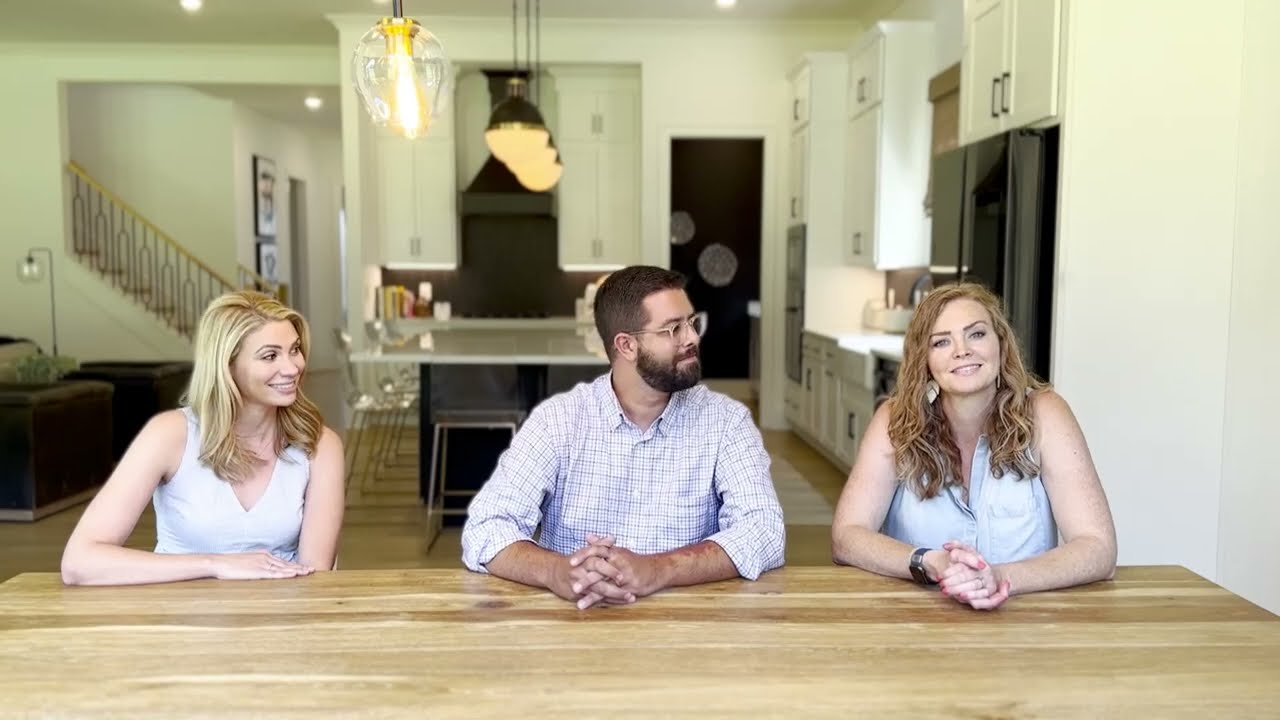The photograph captures three individuals seated at a large, rectangular wooden table, distinguished by its light color, visible wood grain, and knots. The trio consists of two women and one man, all dressed in casual business attire. The man, situated in the center, has short black hair, a black beard, and glasses, and wears a light blue plaid button-up shirt. His hands are interlocked on the table. The woman on the left, with smooth long blonde hair and fair skin, wears a white sleeveless V-neck top. The woman on the right, of a heavier build with long, curly blonde hair falling to her shoulders, wears a sleeveless white shirt, silver earrings, and a wristwatch. 

Both the man and the woman on the left are looking at the woman on the right, who gazes directly at the camera with her hands clasped on the table. The scene is set in a modern kitchen with white cabinetry, a black refrigerator, and a large white marble countertop with a black base. A bar section with chairs is visible behind the trio, and beyond that, the living room furniture and a stairwell in the hallway are discernible. The walls in the background are off-white, contributing to the contemporary aesthetic of the setting.